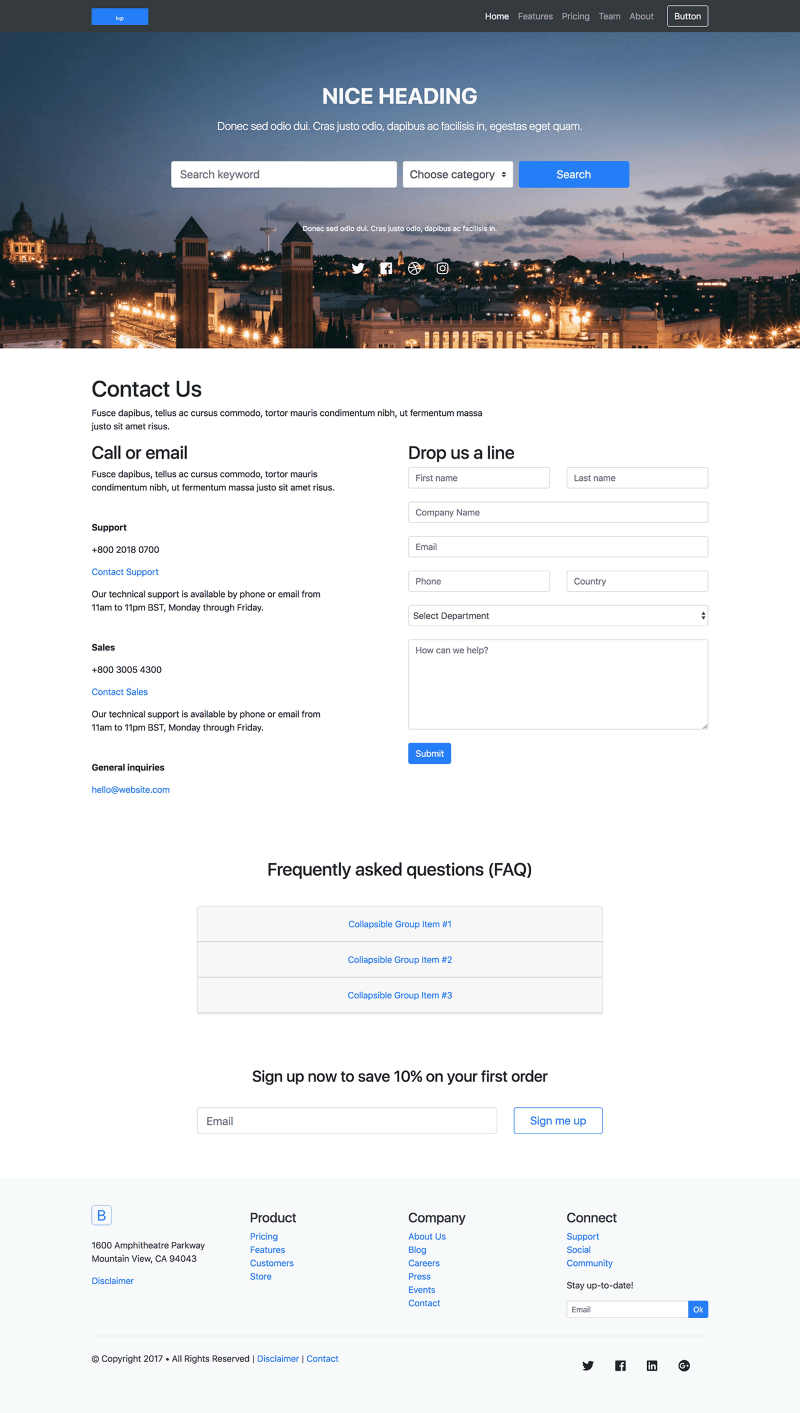The image depicts a full webpage of a website showcasing various sections and features. At the top of the page, there's a black banner with a blue button on the left side. To the right of the button, there are navigation options, including "Home" which is highlighted, "Pricing," and other selections. Adjacent to these is a rectangular button.

In the center of the page, there's a prominent heading that reads "Nice Heading," followed by a line of information consisting of a small, unreadable sentence. Below this, there is a search interface with a field labeled "Search Keyword," a dropdown menu labeled "Choose Category" with arrows for selection, and a blue "Search" button.

The background image beneath these elements appears to be a scenic aerial view of a European city against a clear sky. Below this, there is a "Contact Us" section providing options to call or email, along with a support number and additional contact information.

To the right, there is a "Drop Us A Line" form with fields for first name, last name, email, phone number, and other details. Further down, there's a "Frequently Asked Questions" section with three centered boxes providing various topics. There's also a sign-up box encouraging users to "Sign Up Now to Save 10% on Your First Order," accompanied by an email input field and a "Sign Me Up" button. Lastly, there is additional information on various website areas, highlighted in blue, displayed towards the bottom of the page.